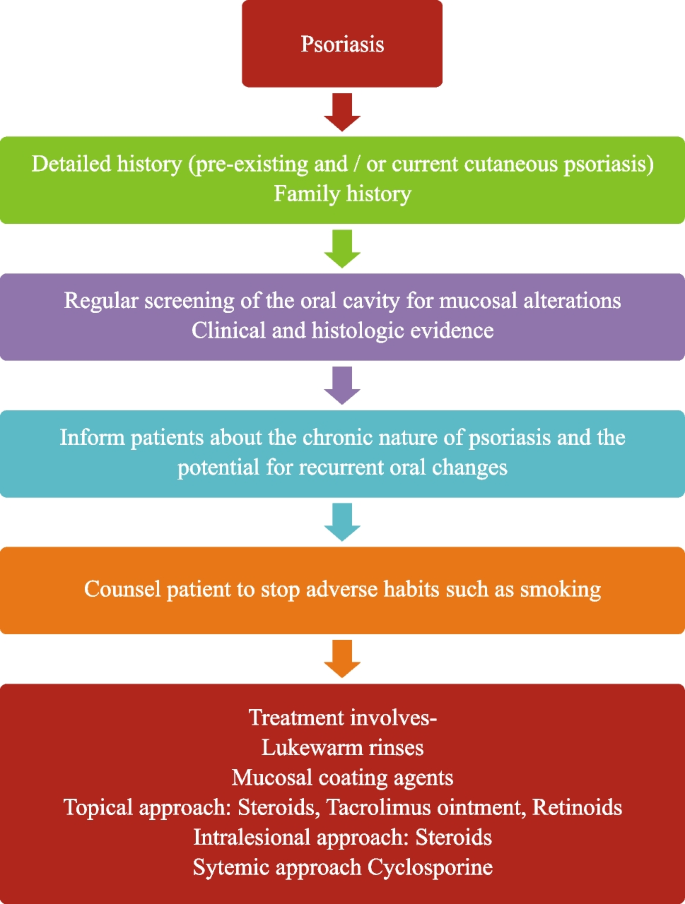The image showcases a flowchart on a white background designed for medical advice related to psoriasis. The flowchart features six colored rectangular boxes connected by arrows that guide the reader from one step to the next in a sequential manner. The top box is wine red and labeled "Psoriasis." The subsequent bright green box provides details on "Detailed history (pre-existing and/or current cutaneous psoriasis, family history)." Next, a purple box states "Regular screening of the oral cavity for mucosal alterations, clinical and histologic evidence." The following blue box informs patients about "The chronic nature of psoriasis and the potential for recurrent oral changes." The orange box advises to "Counsel patients to stop adverse habits such as smoking." The final red box outlines that "Treatment involves lukewarm rinses, mucosal coating agents, topical approaches (steroids, tacrolimus ointment, retinoids), and intralesional or systemic approaches (steroids, cyclosporine).” The flowchart provides a clear and detailed step-by-step guide for managing psoriasis.